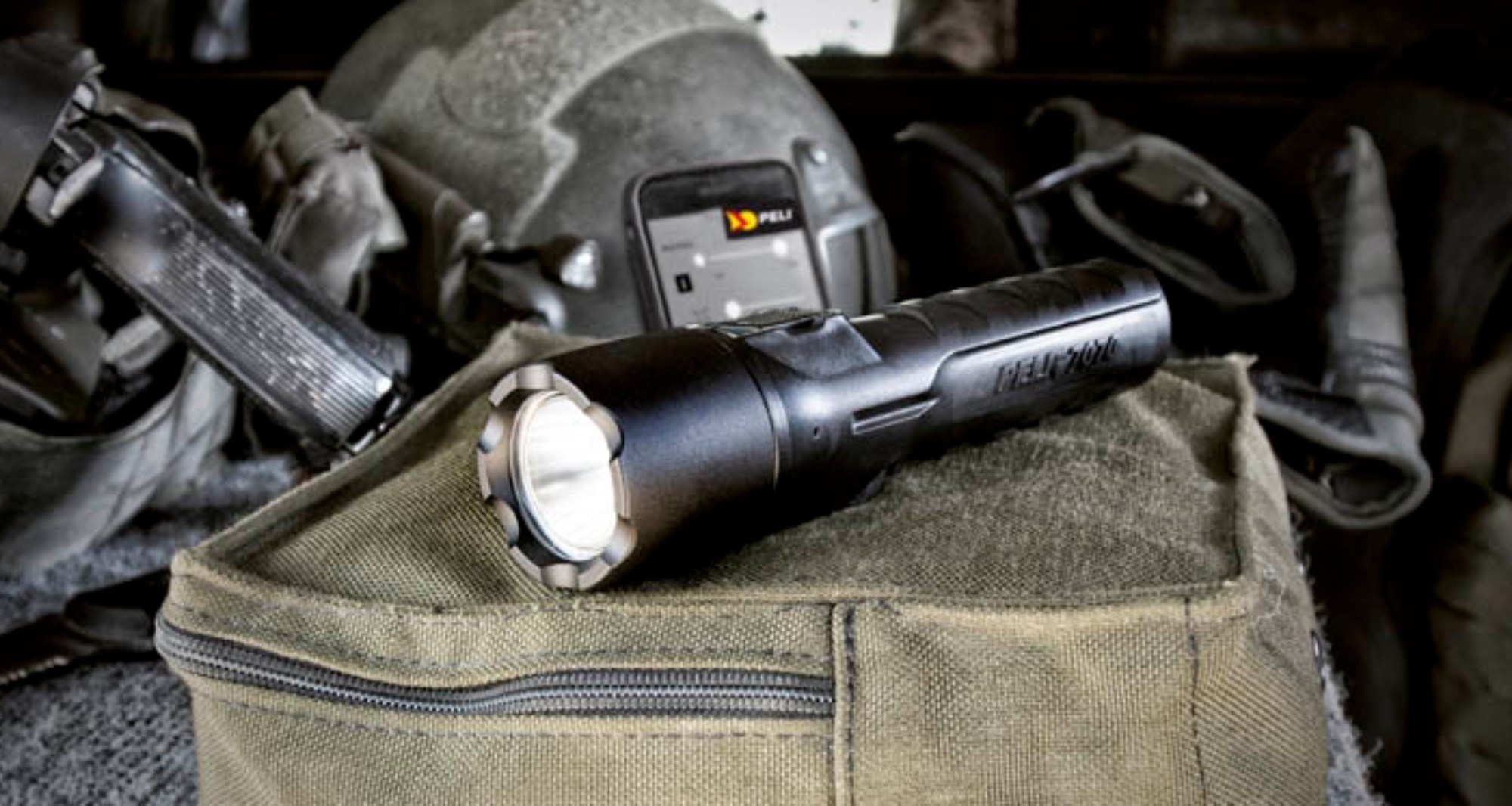This close-up and horizontal photograph features a rugged-looking, industrial black flashlight that is turned on, resting atop a beige or green khaki square canvas bag with a visible side zipper. In the background, slightly out of focus, is a phone with an unreadable app open, resting on what might be a gray helmet tied with cloth. Surrounding these main items are various black and gray objects, scattered haphazardly. Some of these items could be tactical gear or survival tools, possibly used by military or police forces, hinting at a professional, staged setting. The scene is complex and cluttered, with metallic and light-colored items also visible in the periphery.